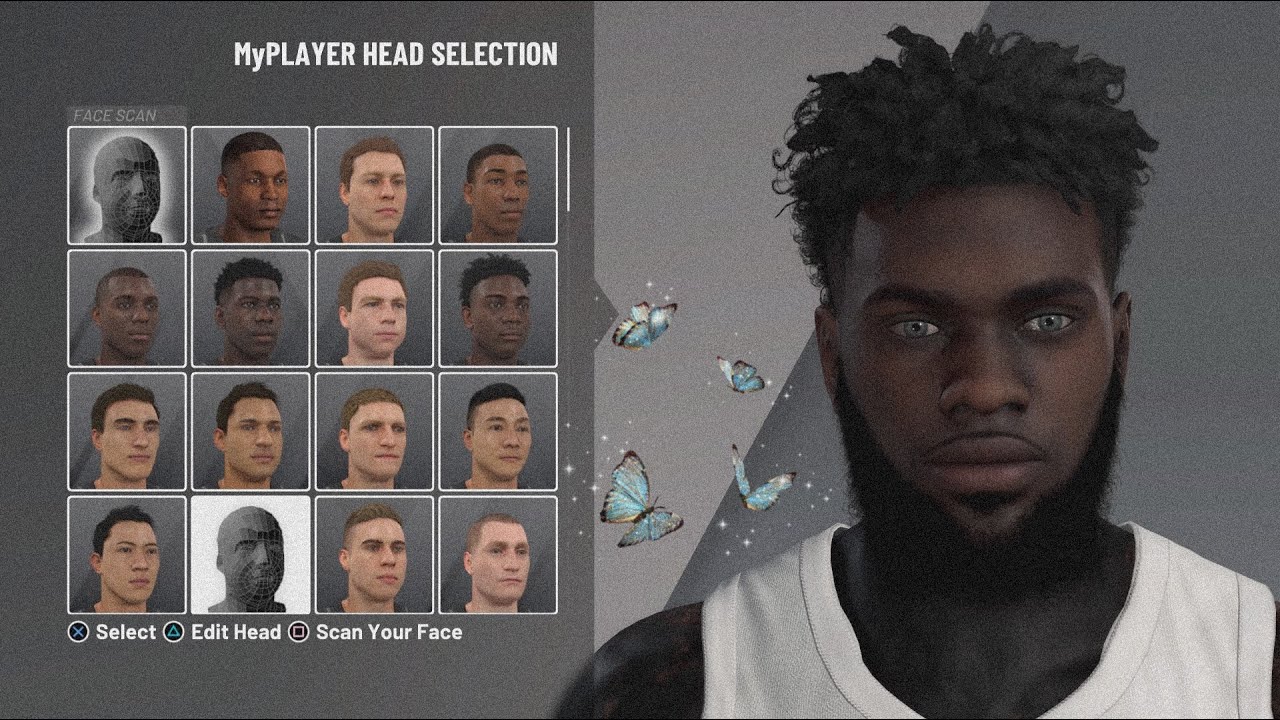In this detailed character creation screen, we observe the interface of a video game allowing for extensive customization. Visible are 16 distinct head models, providing diverse options for the player. Currently, the 14th head model is selected, showcasing a character adorned with birds in their hair and wearing a white vest. To the left of the character, blue butterflies add a whimsical touch to the scene. At the bottom of the screen, options such as "Select," "Edit Head," and "Scan Your Face" are available, offering further personalization. The top of the screen features a label titled "My Player Head Selection," indicating the current customization mode. This visual interface is designed to offer both aesthetic and functional details essential for crafting a unique in-game character.